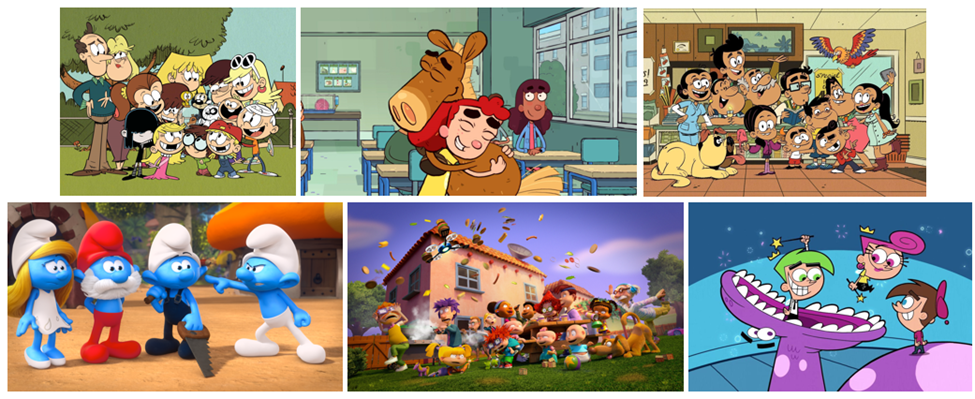The image showcases six cartoon TV show still frames, each capturing a distinct scene. In the top-left panel, the frame features a large family from "The Loud House," assembled together in a grassy field. Adjacent to it, the top-center panel depicts a classroom where a young boy is affectionately hugging a human-like horse while a girl with red hair looks on. The top-right scene portrays a Hispanic family in an indoor setting with an eye-catching bird, displaying vibrant colors of orange, red, and blue, hovering above them. Moving to the bottom row, the bottom-left features CGI Smurfs, including Papa Smurf in red, a blonde female Smurf in a white dress, and two other blue-skinned characters in an outdoor setting. The bottom-center showcases the "Rugrats" cast outside, seemingly engaged in a chaotic yet joyful food fight in a backyard. Lastly, the bottom-right frame from "The Fairly OddParents" shows a fairy with light green hair trapped in the mouth of a purple dinosaur-like creature, alongside another fairy with pink hair and a young boy in a blue room.